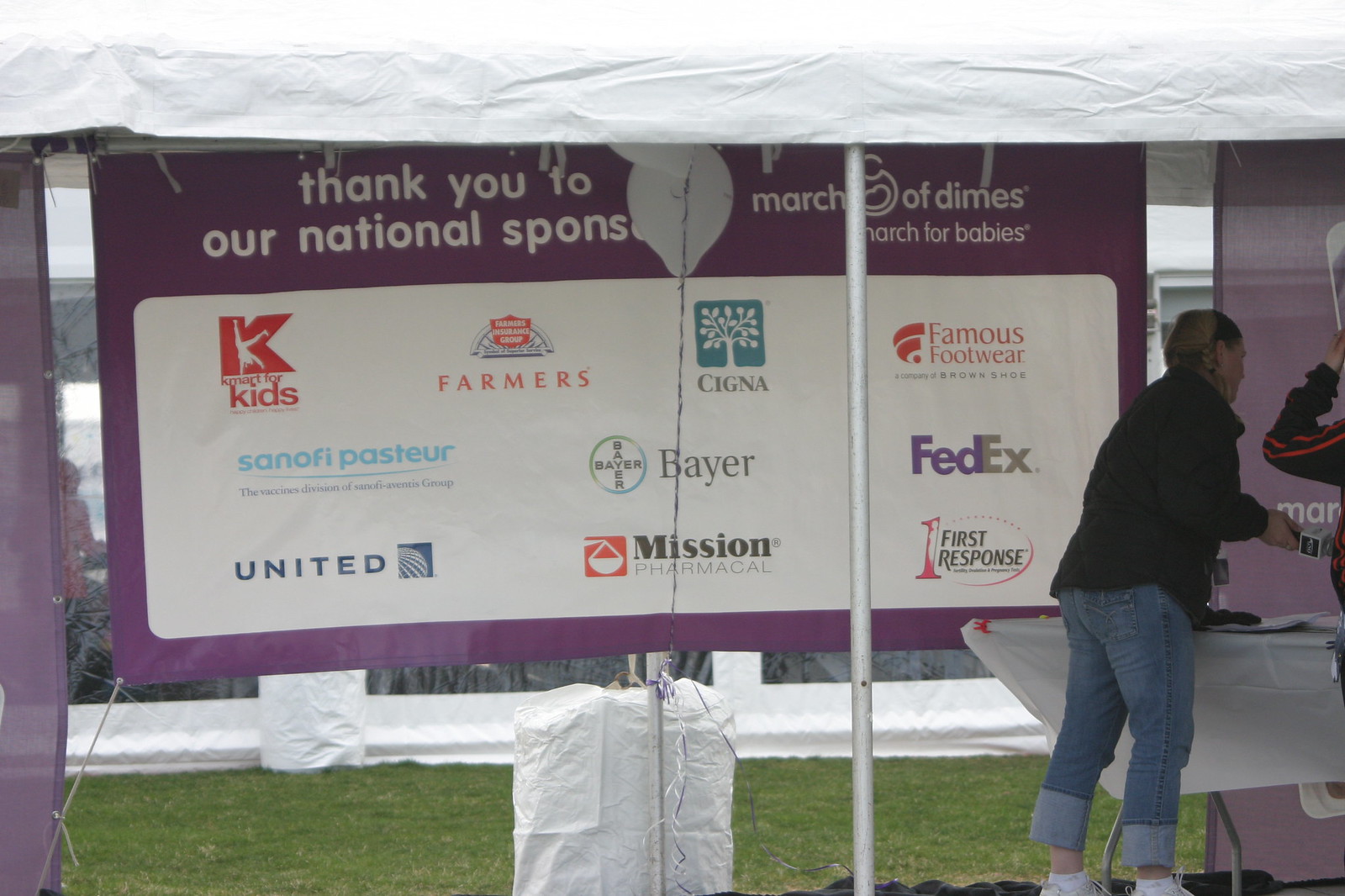The image depicts an outdoor event, possibly under a tent, promoting the March of Dimes' March for Babies campaign. Dominating the scene is a large, purple and white banner hanging from the tent's roof. The top portion of the banner reads "Thank you to our national sponsors," followed by "March of Dimes, March for Babies." The lower section of the banner features a collection of company logos and names such as FedEx, Cigna, Famous Footwear, Farmers Insurance, Kmart for Kids, United Airlines, Mission Pharmaceutical, First Response, Bayer, and Sanofi Pasteur. In the foreground, a woman dressed in a black jacket and jeans stands near the banner. A white table and another woman can be seen under the tent, which has a white overhang supported by a silver pole. The ground is covered in green grass, indicating it's a sunny daytime event.